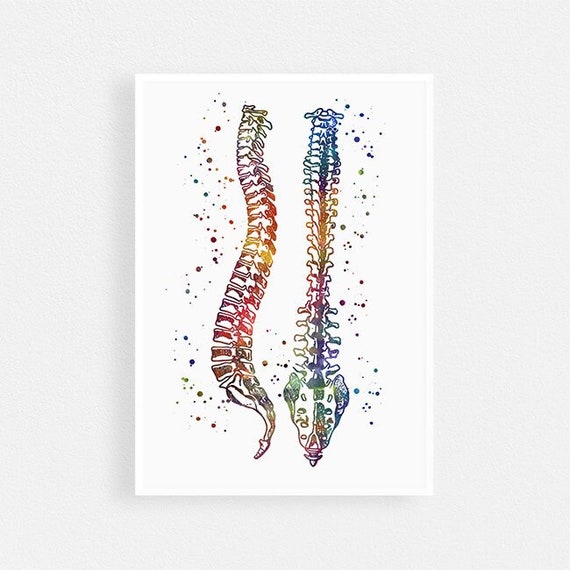The image depicts a vibrant and detailed painting of two spine-like structures set against a white rectangular canvas, positioned vertically on a white plaster wall. The left structure, reminiscent of a snake's tail or a seahorse, is portrayed from a side view, slightly turned to reveal part of its front, and displays a gradient of warm rainbow colors including red, orange, pink, and yellow. This section appears segmented, with scales or vertebrae distinctly separated, and is surrounded by multicolored paint splotches. To the right, the composition showcases a top-down view of a structure resembling a snake's head or a xylophone, accentuated by cool hues of blue, purple, some red, and a touch of orange. This form extends straight up and down, further emphasizing the segmented nature of the depicted skeletal forms. The entire scene is adorned with speckles of rainbow-colored dots, adding to its dynamic and vividly artistic presentation, and creating an almost framed effect within the photograph.